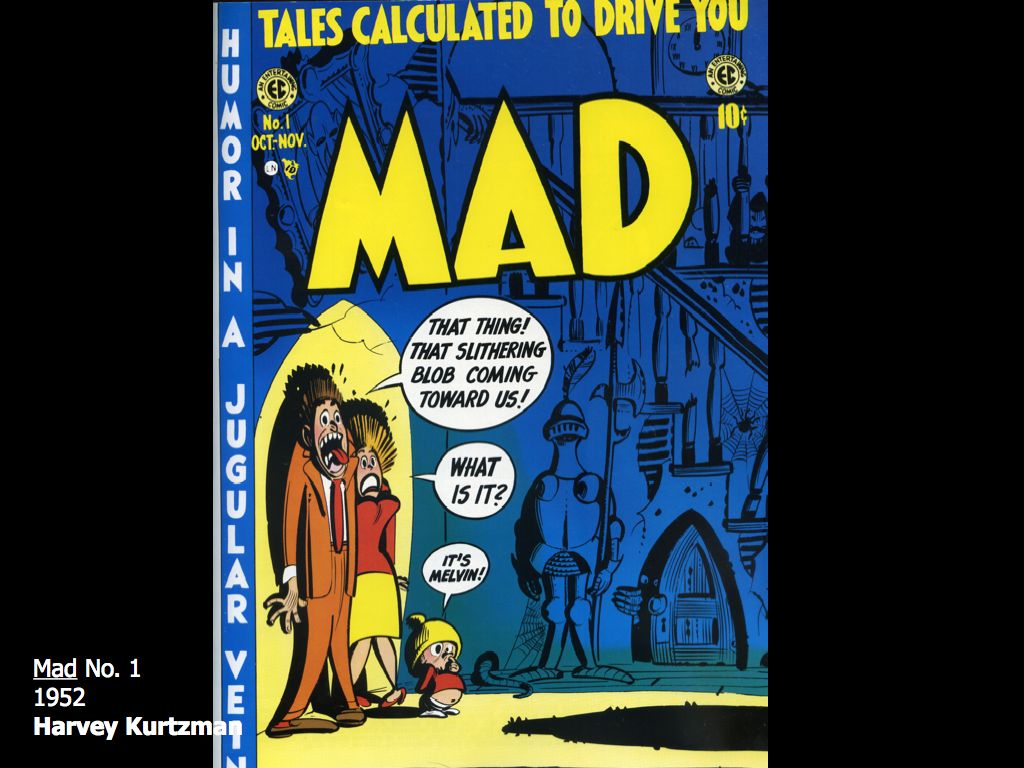This image showcases the cover of the first edition of MAD Comic Book from 1952, illustrated by Harvey Kurtzman. The title "M.A.D." is prominently displayed in large yellow letters at the top, with the subtitle "Tales Calculated to Drive You Mad" beneath it. The setting appears to be a rundown, creepy house, with an intricate arrangement of items like a staircase, a knight’s armor display, and a small wooden door under the stairs. The comic cover's backdrop is primarily blue, accentuated with black ink illustrations and highlighted sections in white, suggesting light entering the room from an opening door. 

Central to the cover are three frightened family members—an orange-suited man with a red tie, a woman in a red top and white skirt, and a small child in red attire with a yellow hat—backed against a wall. Their expressions convey terror, emphasized by their open mouths and the man’s exclamatory speech bubble, "That slithering blob coming towards us!" The woman echoes, "What is it?" while the child identifies, "It’s Melvin," implying Melvin is a character integral to MAD's identity. A black blob is depicted creeping towards them from the floor. The tagline, "humor in a jugular vein," runs down one side of the cover. The comic's price is marked at ten cents, a nostalgic nod to its era, and the bottom left corner notes, "Mad Number One, 1952, Harvey Kurtzman."